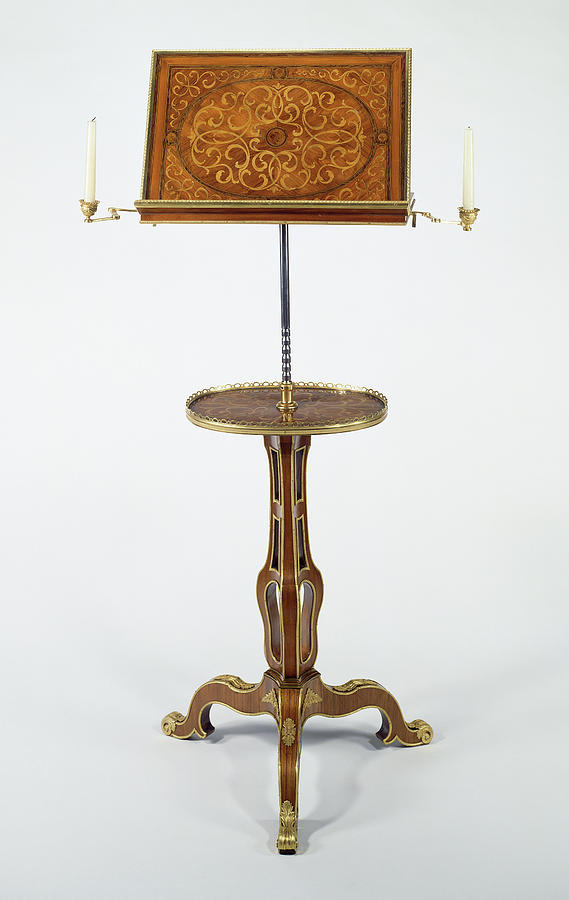The image features a close-up of an antique music stand with a historic and intricate design. The top portion is a brown rectangle adorned with beige, squiggly line patterns and random round designs. A gold-colored stick hangs out with a white tapered candle on either side. Below, there's a shiny, dark-colored stick and a bronze, circular plate. The lower portion of the stand is thick, brown, and black with a bulging design. The stand rests on three curved, brown legs with gold trim. The material appears to be a mix of wood with gold, brass, or copper accents. The music stand is set against a gray background, centered in the image, which is bright and clear with natural lighting. The overall appearance suggests a historic, possibly French, origin.